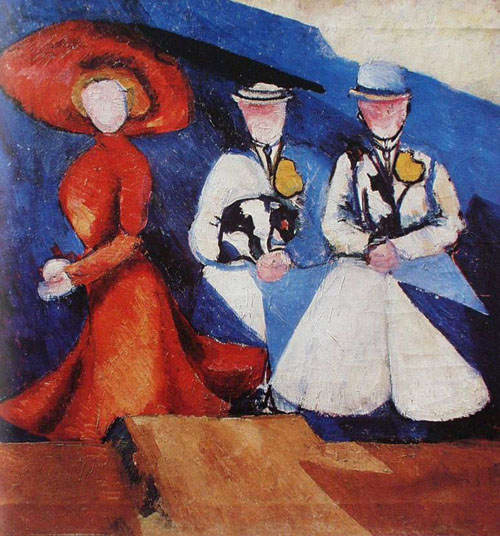This is an oil painting titled "Three Female Figures" by Alexandra Ekster, created in 1910. The painting, executed in an abstract impressionist style, is presented in a square format. The scene features three faceless figures, emphasizing a sense of anonymity and abstraction. The most prominent figure on the left side is a woman dressed in a lavish red ensemble, including a wide-brimmed hat and a long, flared dress that fits tightly at the torso before cascading outward. She has short, auburn hair and is depicted in profile, looking over her left shoulder towards the viewer. 

To her right stand two figures, also faceless and dressed in white. Both wear wide-brimmed white hats, with one figure sporting a blue band and a tie under the chin. One of these figures appears slightly larger and closer to the viewer, and their white overcoat flares out in two petal-shaped sections. The background comprises a mix of dark blue and white shades, while the foreground features a brown, almost wooden-like texture, enhancing the depth and complexity of the piece. The color palette includes prominent reds, whites, browns, grays, blacks, dark blues, peaches, and touches of yellow, devoid of any text. The figures and background meld together in a harmonious blend of color and form, characteristic of abstract impressionism.